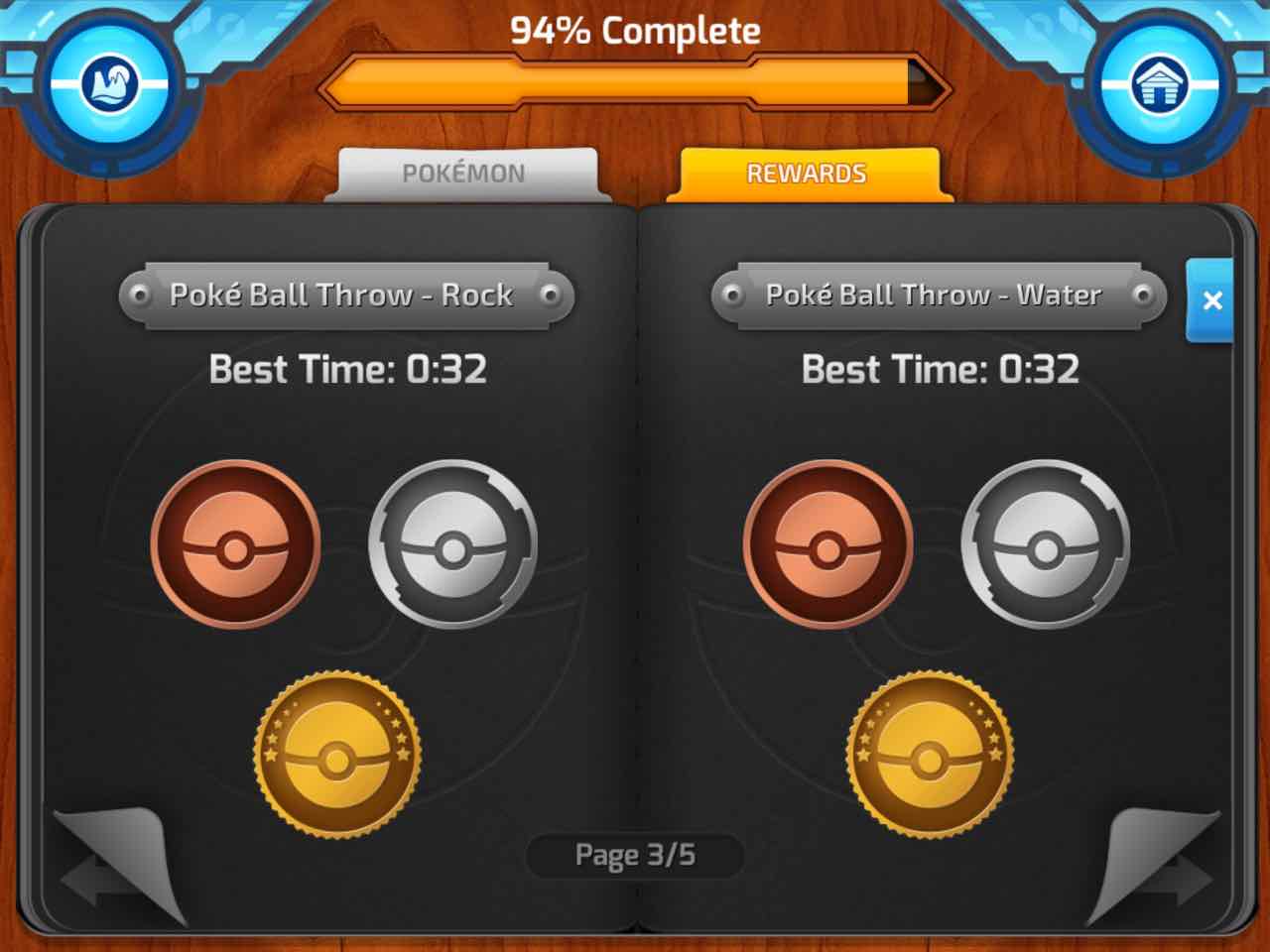The image is a screenshot from a Pokémon game, captured in a rectangular frame. The background features a wooden table pattern. In the upper left and right corners are light blue circles outlined with dark blue. The left circle contains an image resembling mountains with a sun behind them, while the right circle has a small white house icon inside. At the top center, white text reads "94% complete," positioned above an orange progress bar that is nearly full.

Below the progress bar is an open black notebook displaying two pages. The left page has a gray tab at the top labeled "Pokémon" in white letters. Beneath this, there is a gray box with the text "Pokéball Throw Rock." Below that is "Best Time: 32 seconds," followed by three symbols representing different Pokéballs: a bronze, a silver, and a gold Pokéball.

The right page features a yellow tab at the top labeled "Rewards" in white letters. It also displays "Pokéball Throw Water," the same "Best Time: 32 seconds," and the same three Pokéball symbols as the left page. At the bottom center of the notebook, small text indicates "Page 3 of 5."

In the lower left and right corners of the notebook, arrows indicate the option to navigate back and forth between pages.